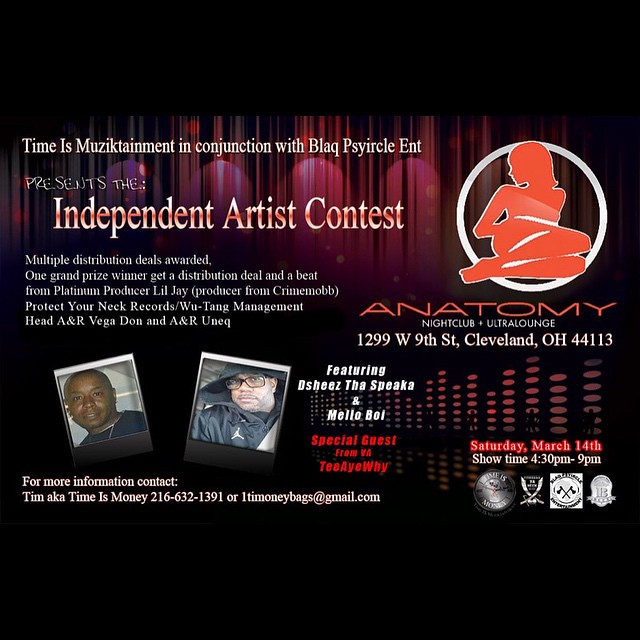The image is an advertisement from Anatomy Nightclub promoting an Independent Artist Contest. The advertisement, by Time is Musictainment in conjunction with Black Psyircle Ent, announces multiple distribution deals to be awarded, with one grand prize winner receiving a distribution deal and a beat from platinum producer Lil J, known for his work with Crime Mob. Additional notable figures included are Protect Ya Neck Records/Wu-Tang Management's Head A&R Vega Dawn and A&R UNEQ. The flyer features photos of two black men alongside an email address and phone number for further contact. On the right side, a red silhouette of a woman posed seductively emphasizes the venue, Anatomy Nightclub Ultra Lounge, located at 1299 West 9th Street, Cleveland, Ohio, 44113. The event is scheduled for Saturday, March 14th, with showtime from 4:30 PM to 9:00 PM. For more information, contact him at 216-632-1391 or one-time-ti-moneybags at gmail.com.